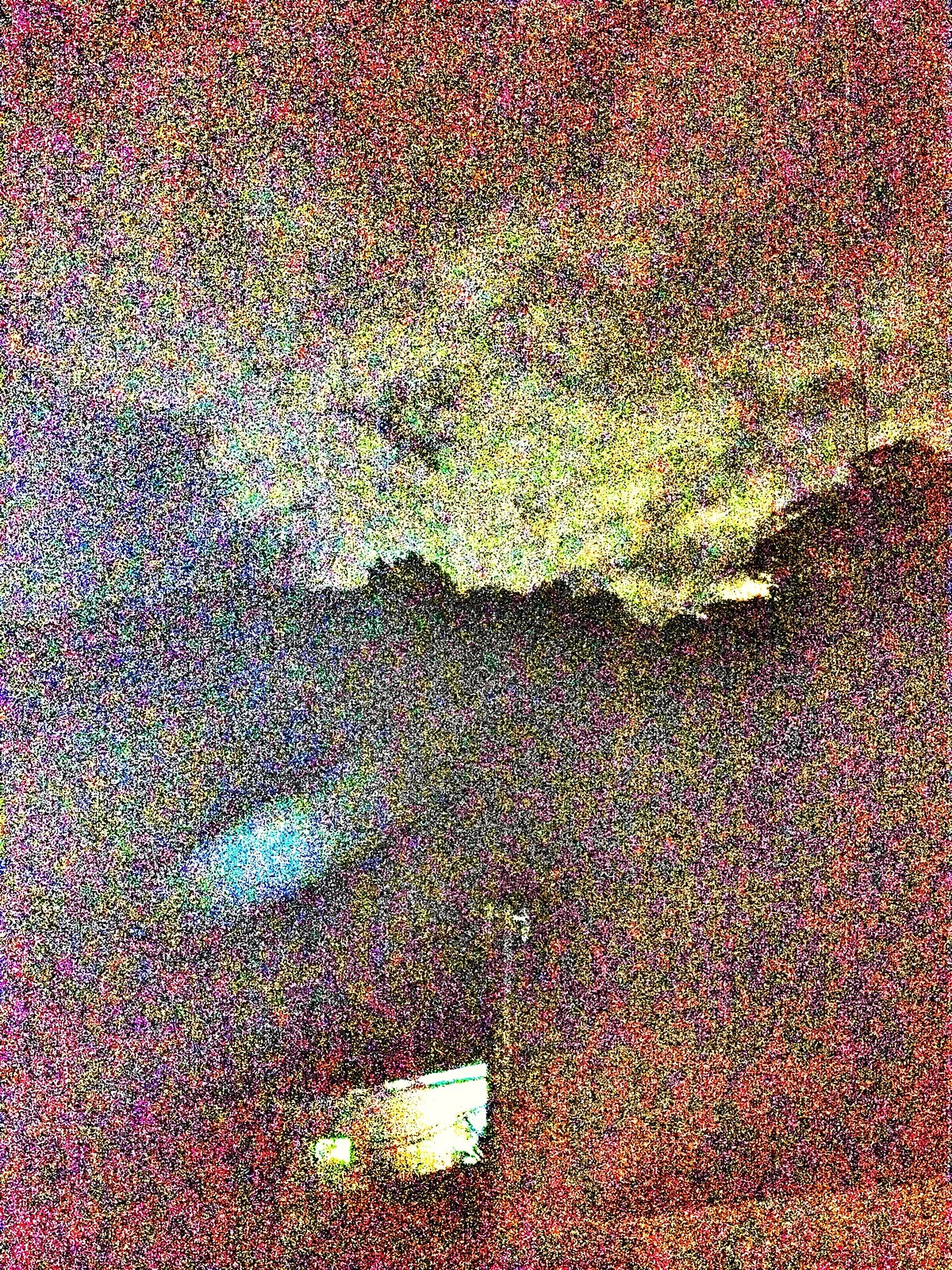This image is an exceptional example of pointillism, where the entire composition is created from countless small dots of various colors. The upper portion of the image features a sky rendered in a gradient of pink and purple dots, transitioning into a deeper purple as you move downward. Below this section, the dots form splotches of ivory with gray interspersed, indicating the beginning of a hilly horizon adorned with faintly discernible trees. The lower half of the image presents a darker array of pink and purple dots, accented with lighter tannish dots. At the very bottom, a somewhat unclear white rectangle breaks the dot pattern, creating a semi-solid shape. To the right of this rectangle stands a pole with an indistinct object at its top. Additionally, a cluster of light blue dots appears above this section, slightly to the left, adding another layer of complexity to the scene.